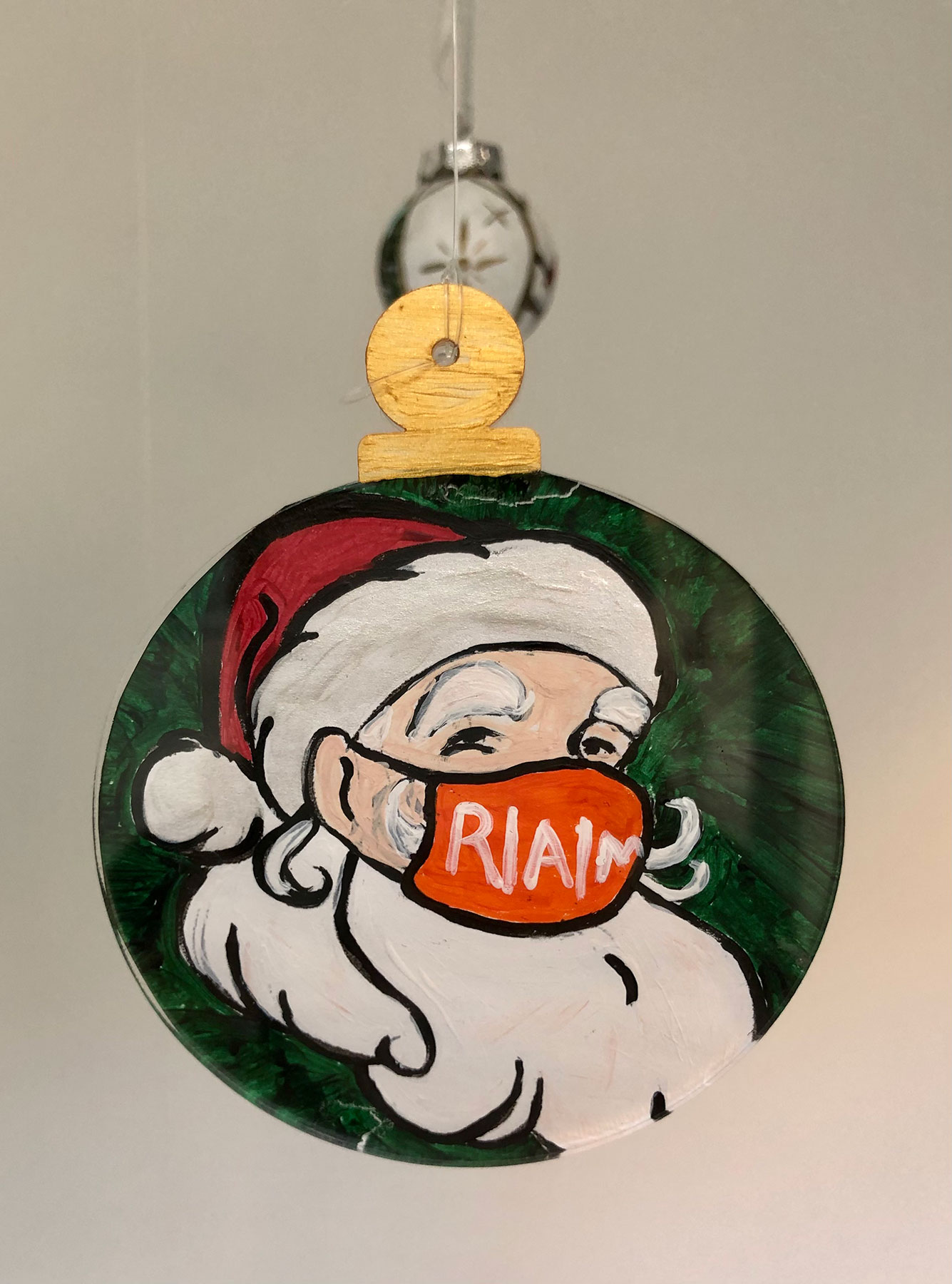The image is a detailed closeup of a handmade Christmas ornament carved from wood and painted. The ornament is flat and circular with a green-painted background and features a hand-painted depiction of Santa Claus. Santa is adorned in his classic red hat with white trim, fluffy white eyebrows, and a white beard. Notably, he is wearing a mask over his nose and mouth, which is painted orange and bears the text "R.I.A.L.M." or "R.I.A.I.M." (the exact sequence is unclear but is an important detail). The ornament hangs by a string attached through a hole at the top, which is plain and unpainted, revealing the natural yellow wood. In the background, there is another store-bought ornament with a silver top and a small white snowflake design.